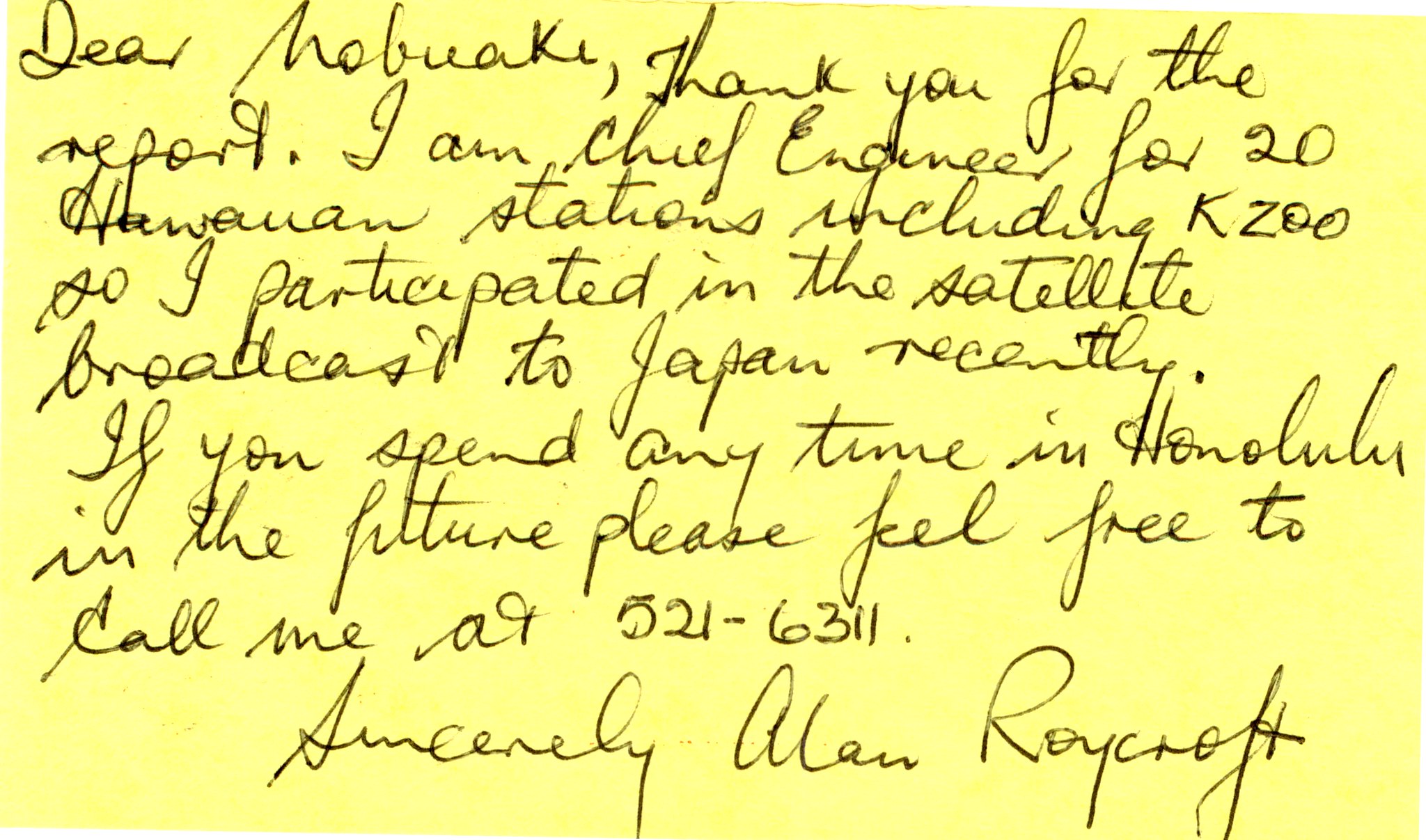The image is a digital screenshot of a handwritten letter on a light yellow, canary-like piece of paper. The note is from Alan Roycroft, the chief engineer for 20 Hawaiian stations, including KZOO. In clear cursive writing with black ink, the letter reads: "Dear Mabake, Thank you for the report. I participated in the satellite broadcast to Japan recently. If you spend any time in Honolulu in the future, please feel free to call me at 521-6311. Sincerely, Alan Roycroft." The letter is a short paragraph in length and serves as a QSL note, likely sent to someone named Mabake who might be in Japan.